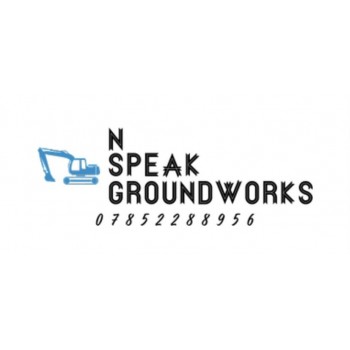The logo for InSpeak Groundworks is set against a white background and prominently features solid blue and black colors. At the top of the vertically aligned text, the letter 'N' appears in black. Directly underneath is the word "speak" and below that is "groundworks," both in matching black text. The text is organized in a vertical stack, creating an arrangement that reads as "NSG" from top to bottom. Below the words "InSpeak Groundworks" is a set of digits, presented in smaller print, that reads 07852288956, which likely serves as a contact number. To the left of the text is a blue silhouette of an excavator, characterized by a body on treads with an arm and claw extending from it. The excavator image is minimalistic and quite small compared to the textual elements of the design. The overall composition is clean and focused on the business identity and contact details.